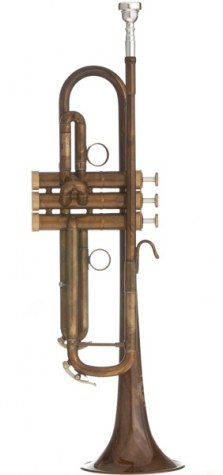The image features an old-fashioned, vertically positioned trumpet against a white background. The trumpet, rendered in a somewhat artistic and faded style, appears as aged brass or dulled bronze. It includes a chrome or silver-gold mouthpiece pointing upwards, contrasting with the rest of the instrument's muted tone. The body of the trumpet is adorned with three buttons on the right side, and it is unclear whether this is a real trumpet or a detailed drawing of one. The instrument shows signs of wear, hinting at rust and an unpolished surface. Additional details such as a hook and small rings are visible, likely intended for holding and maneuvering the instrument. The overall presentation of the trumpet is simple yet detailed, emphasizing its vintage and well-used appearance.